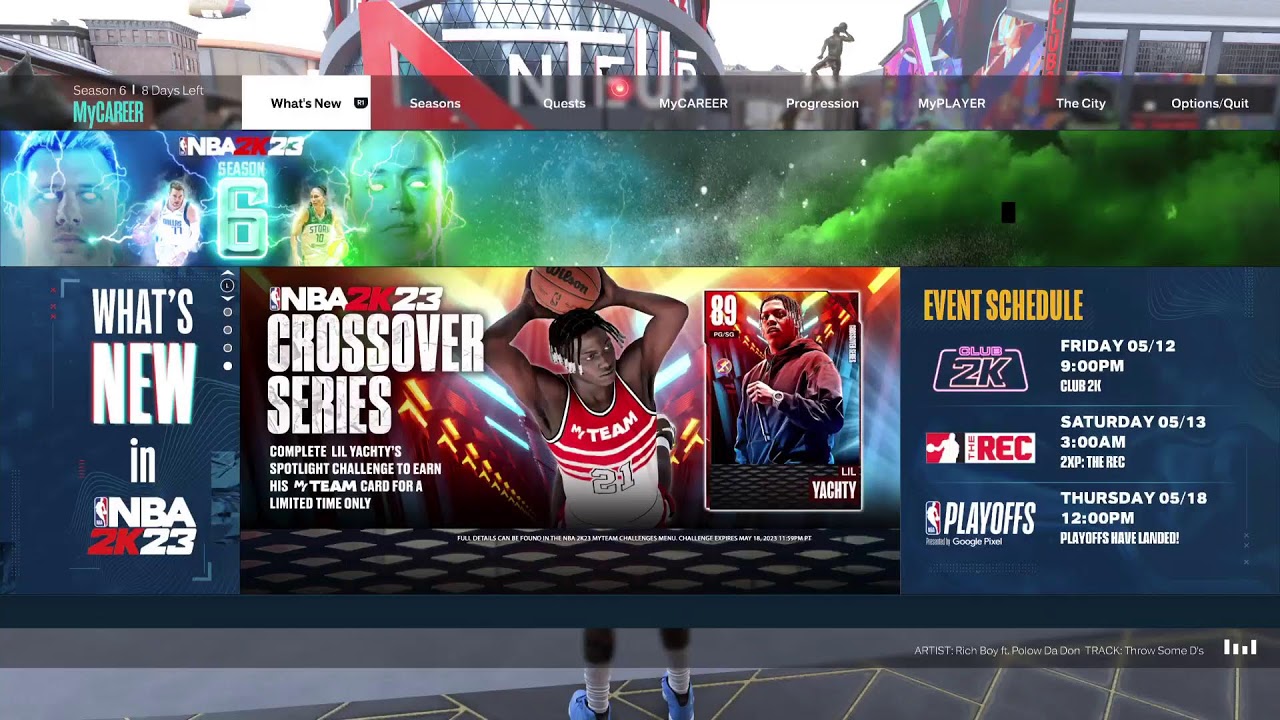The image depicts a webpage designed for accessing NBA sporting events, specifically related to the NBA 2K23 game. The top of the webpage features a navigation bar with various options including "What's New," "Seasons," "Quests," "My Career," "Progression," "My Player," "The City," "Options," and "Quit." 

At the center of the page is a themed graphic prominently displaying the text "NBA 2K23 Crossover Series." The graphic features a dynamic image of a basketball player mid-action, about to shoot a ball into the hoop. 

On the right-hand side of the page, there is an event schedule detailing upcoming events: "Club 2K" scheduled for Friday, December 5th at 9pm, "The REC" available on Saturday, December 13th at 3am, and "Playoffs" set for Thursday, May 18th at 12pm.

Additionally, a panel on the left side of the image highlights the segment "What's New in NBA 2K23." Overall, the entire webpage is focused on NBA-related content, with various features and updates pertaining to the NBA 2K23 game.